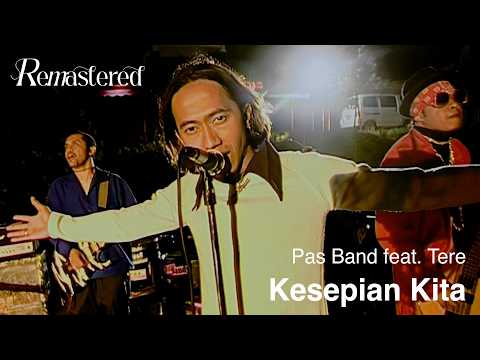This photograph captures an Asian rock band performing outdoors, likely at an outdoor venue at night. The lead singer, who has shoulder-length dark hair, stands front and center wearing a white shirt with a black collar, extending his arms in a cross pose while singing into a microphone positioned slightly below his mouth. To the singer's right, a guitarist is seen playing a black and white animal print design guitar, dressed in a blue buttoned shirt and black pants. To the singer's left, the bass player is distinguishable in a red shirt, red bandana, black hat, and black sunglasses. Behind the band, although the drummer is obscured by the singer, the drum set is visible along with some amplifiers. The backdrop features a parked truck, shrubs, grass, trees, and a parking lot light, indicating that the performance is taking place outside.